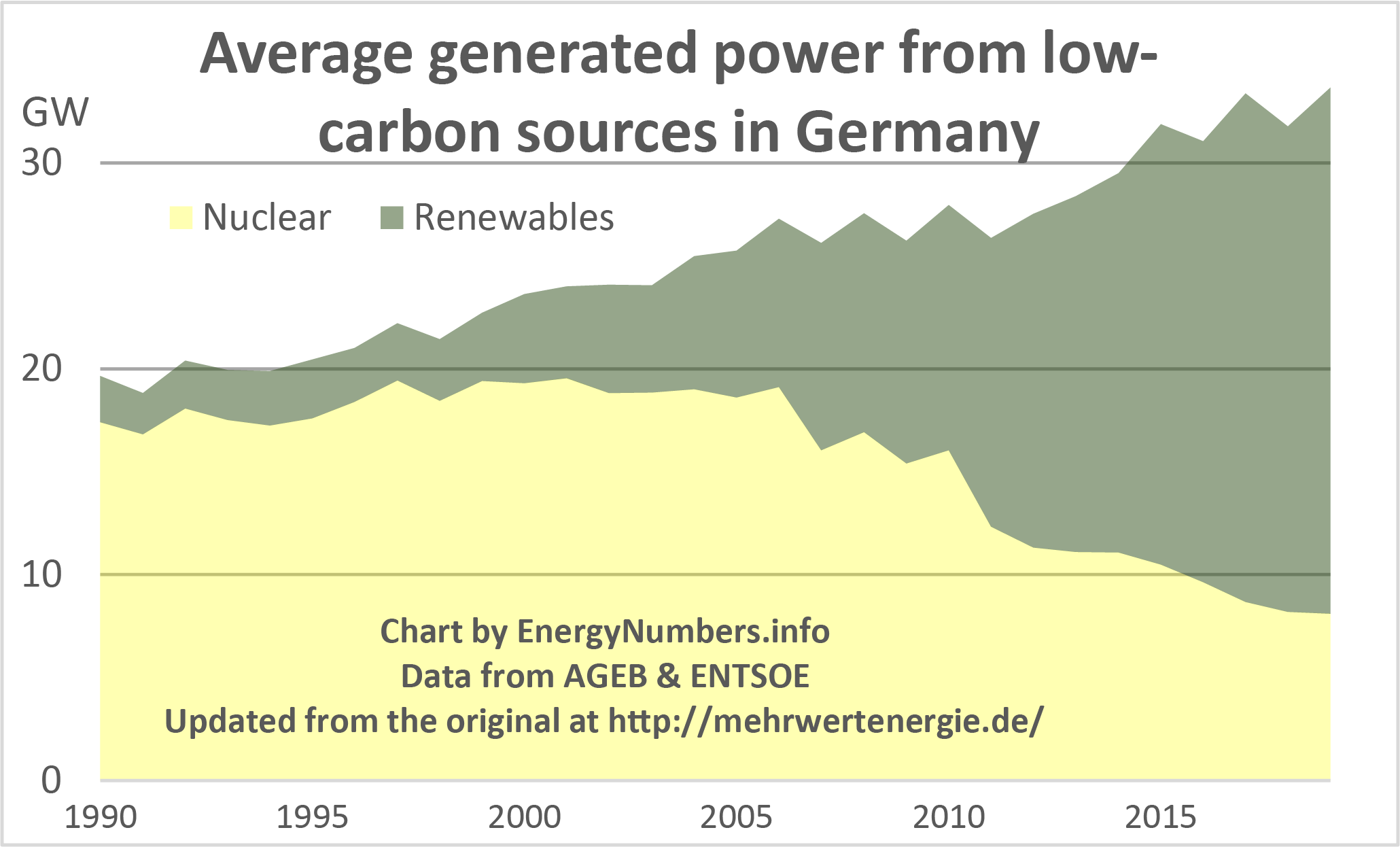The chart titled "Average Generated Power from Low Carbon Sources in Germany" illustrates the progression of power generation from low-carbon sources over time. The graph features angular sections resembling mountain peaks, segmented by color to represent different power sources. 

The yellow segment at the bottom of the graph signifies nuclear power, while the olive-green segment above it represents renewable energy. The vertical axis, measuring power output in gigawatts (GW), starts at zero and increments through 10, 20, and 30 GW. 

The horizontal axis lists specific years: 1990, 1995, 2000, 2005, 2010, and 2015, documenting the changes in power generation over the decades. 

In the early 1990s, nuclear power (yellow) contributed significantly to Germany's low-carbon energy mix. However, a noticeable decline in nuclear power usage begins around 2010. In contrast, the share of renewable energy (olive green) sees consistent growth, eventually dominating the graph by 2015, indicating a significant transition towards renewables in Germany's energy landscape.